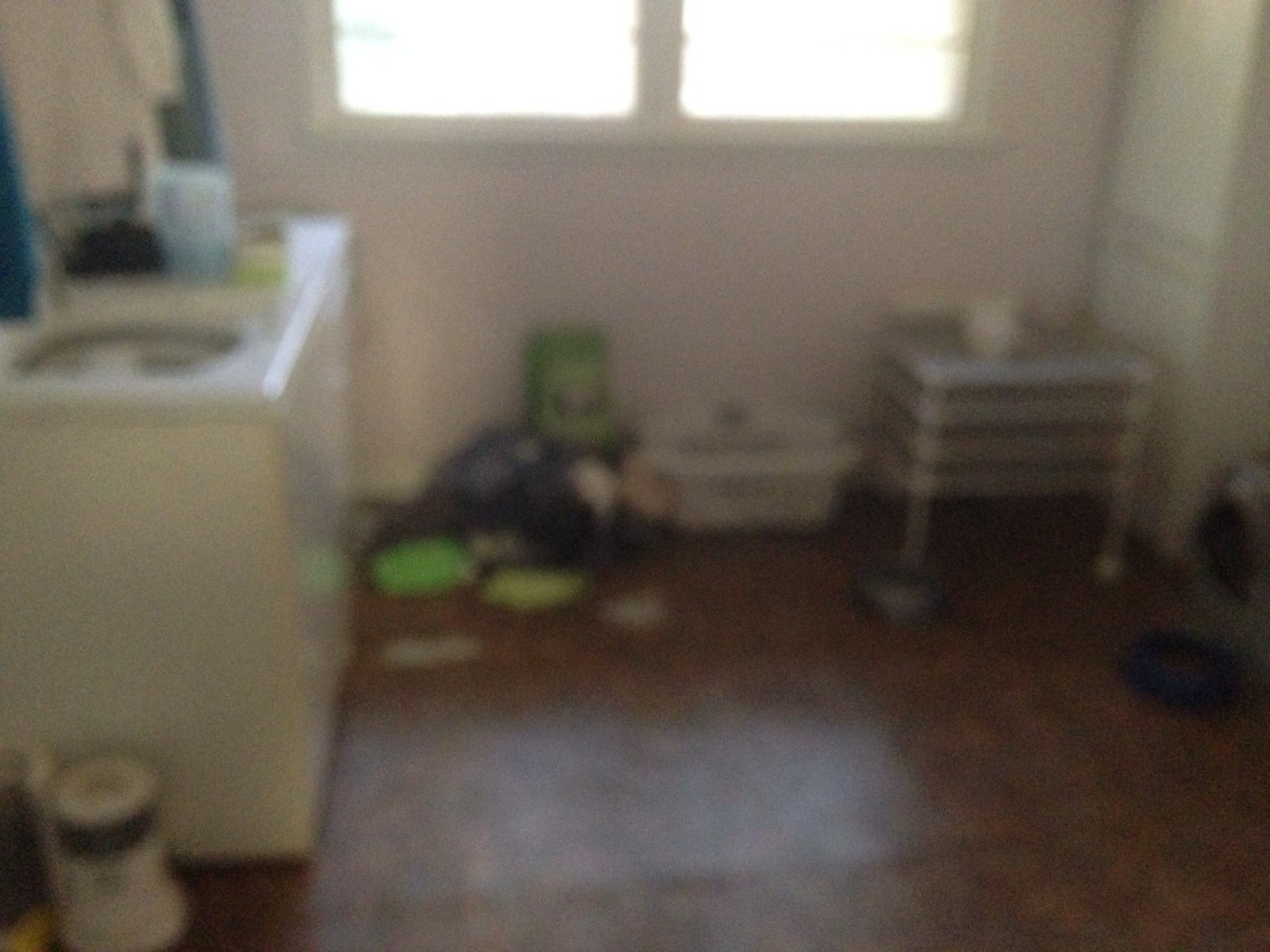This blurry photograph captures the interior of a laundry room with a brown linoleum floor. On the left side, there's a white washing machine with its lid open, revealing the tub inside. Adjacent to the washing machine is a white dryer, which has a blue soap bottle and a small green box on top of it. A roll of paper towels seems to be on the floor in front of the washer. In the center of the image, there's a white laundry basket and a pile of clothes that include blue, green, and yellow items. Next to the basket, there appears to be a gray box with wheels. Up towards the top of the picture, two wide windows allow natural light to flood in. To the right, a tall tan cabinet is visible, and there may be stacked black boxes on the floor beneath the windows. A white drying rack is also mentioned to be near the pile of clothes.